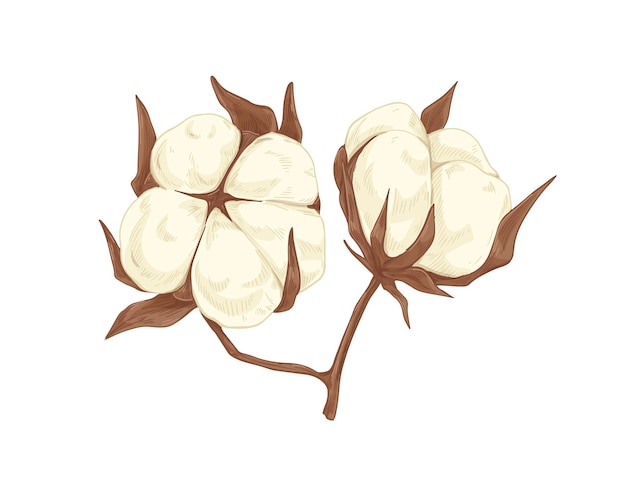This is a detailed depiction of a delicate, white flower set against a pure white backdrop, drawn with color pencils or digitally rendered in a 2D format. Central to the image is a slender stem sprouting from the bottom middle and quickly branching into a Y-formation. Each branch supports a large, fluffy cotton bud that is meticulously folded into five triangular sections converging towards a star-shaped, brown center, creating a dumpling-like appearance. The cotton buds are flanked by sharp, pointed, rippled brown leaves that seem to encase them protectively, with each bud facing opposite directions—one towards the left center and the other towards the right. Notably, one bud appears to be further divided into four distinct sections. Behind the cotton, brown leaves are subtly integrated, reinforcing the plant's textured, natural look. The overall simplicity of the plain white background accentuates the intricate details and contrasts of the flower's structure, making it a visually compelling piece.